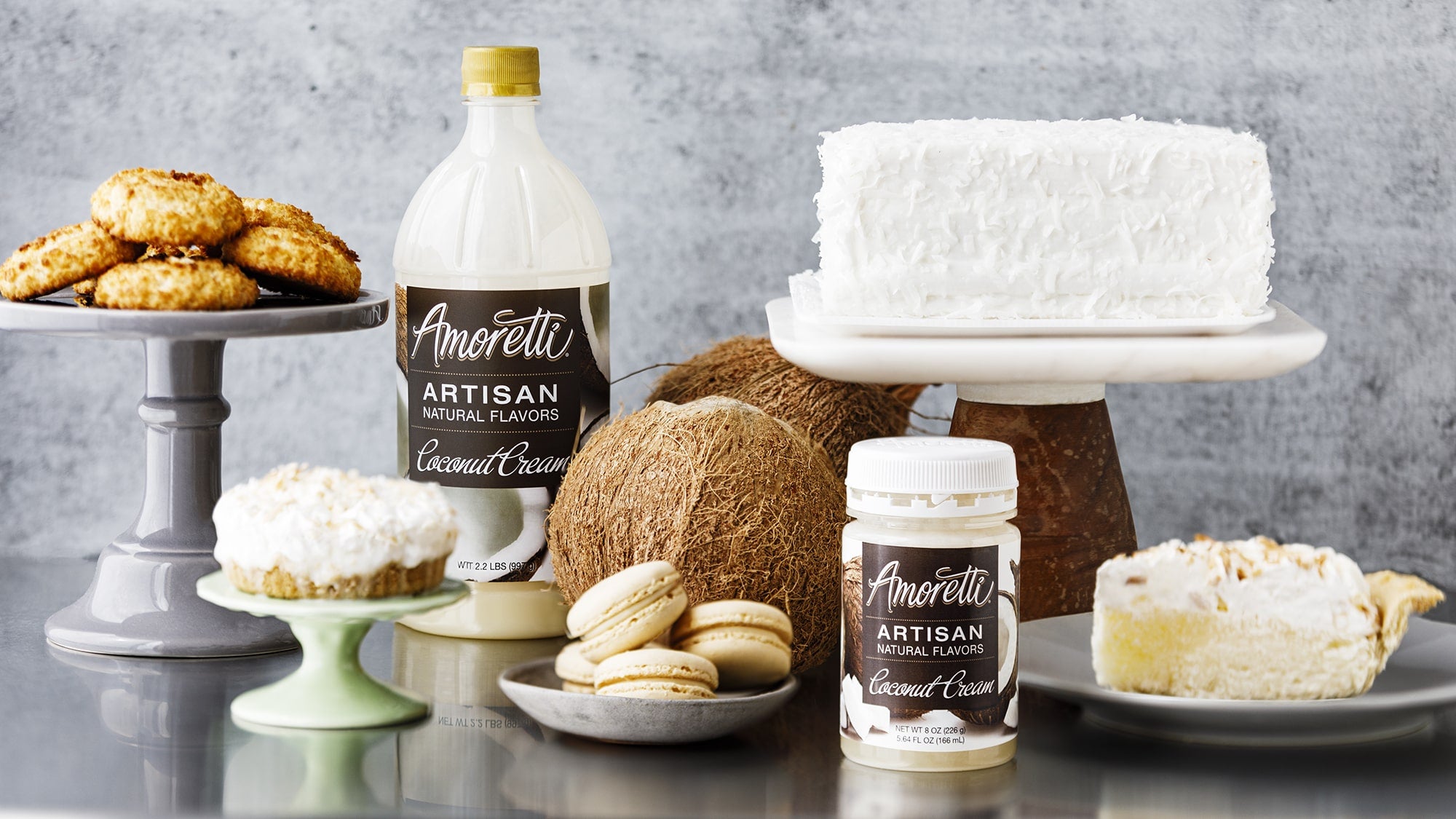This professional food photograph, likely taken by a food blogger, captures an exquisite coconut-themed spread against a gray stone wall. On a shiny, gray-colored surface, various coconut-based treats are displayed, presenting a captivating array of textures and forms. 

To the left sits a gray ceramic pedestal holding a stack of golden brown coconut macaroons. Adjacent to it, a green plate on a matching stand cradles a decadent cream pie, its smooth coconut-infused filling lustrously gleaming under the lighting. 

Central to this arrangement, a sizable white plastic bottle with a golden cap bears a label that reads "Amoretti Artisan Natural Flavors, Coconut Cream," alongside an evocative image of a halved coconut. Nestled next to it is a smaller, peanut butter jar-lookalike container of the same coconut cream, further supporting the cohesion of the theme.

Enriching this tableau, two authentic, brown hairy-skinned coconuts are positioned amidst other culinary delights. A creative white ceramic plate with a brown pillar base showcases a rectangular slab of white cream cake, capturing the essence of simplicity and elegance.

On yet another plate, glossy gray in color, lies another coconut cream dessert, hinting at a luxurious and rich flavor profile. A small gray plate nearby holds a slice of pastry, likely brimming with coconut goodness.

This meticulously arranged setting, with its harmonious blend of natural and crafted elements, highlights the versatility and intricate appeal of coconut as a key ingredient in both traditional and contemporary culinary creations.